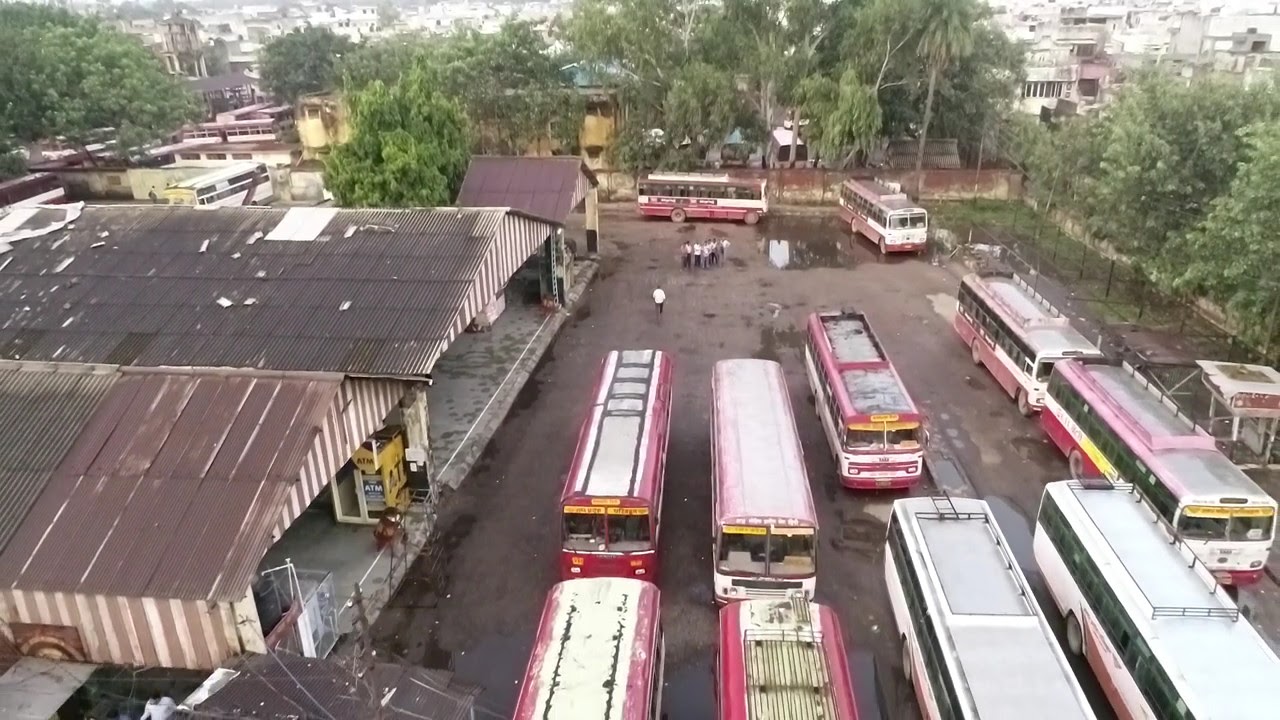The photograph depicts a bustling bus depot, featuring 11 large city buses parked side by side in an organized grid formation. These buses are primarily white with striking red and yellow accents and distinct, school bus-like windows. The parking lot is surrounded by towering trees with long, flowy leaves, casting a green canopy over the area. Adjacent to the parking lot is a weathered, industrial warehouse with rusted, corrugated tin walls and triangular roofs; an ATM is situated against the wall of this large garage structure on the left. The dark gray asphalt of the parking area contrasts with the vivid colors of the buses.

In the center of the image, a group of men wearing white t-shirts stands gathered near the buses, adding a human element to the otherwise industrial scene. The depot is enclosed by a dark fence and a red and white wall on the perimeter. Beyond this, the image expands to reveal a dense metropolitan skyline composed of closely packed, mostly white buildings that might be commercial or residential. The entire scene exudes a slightly damp, humid atmosphere, as if it has just finished raining. The surrounding trees, some with brown and yellowish leaves, intersperse among the distant buildings, hinting at an urban area interwoven with greenery.